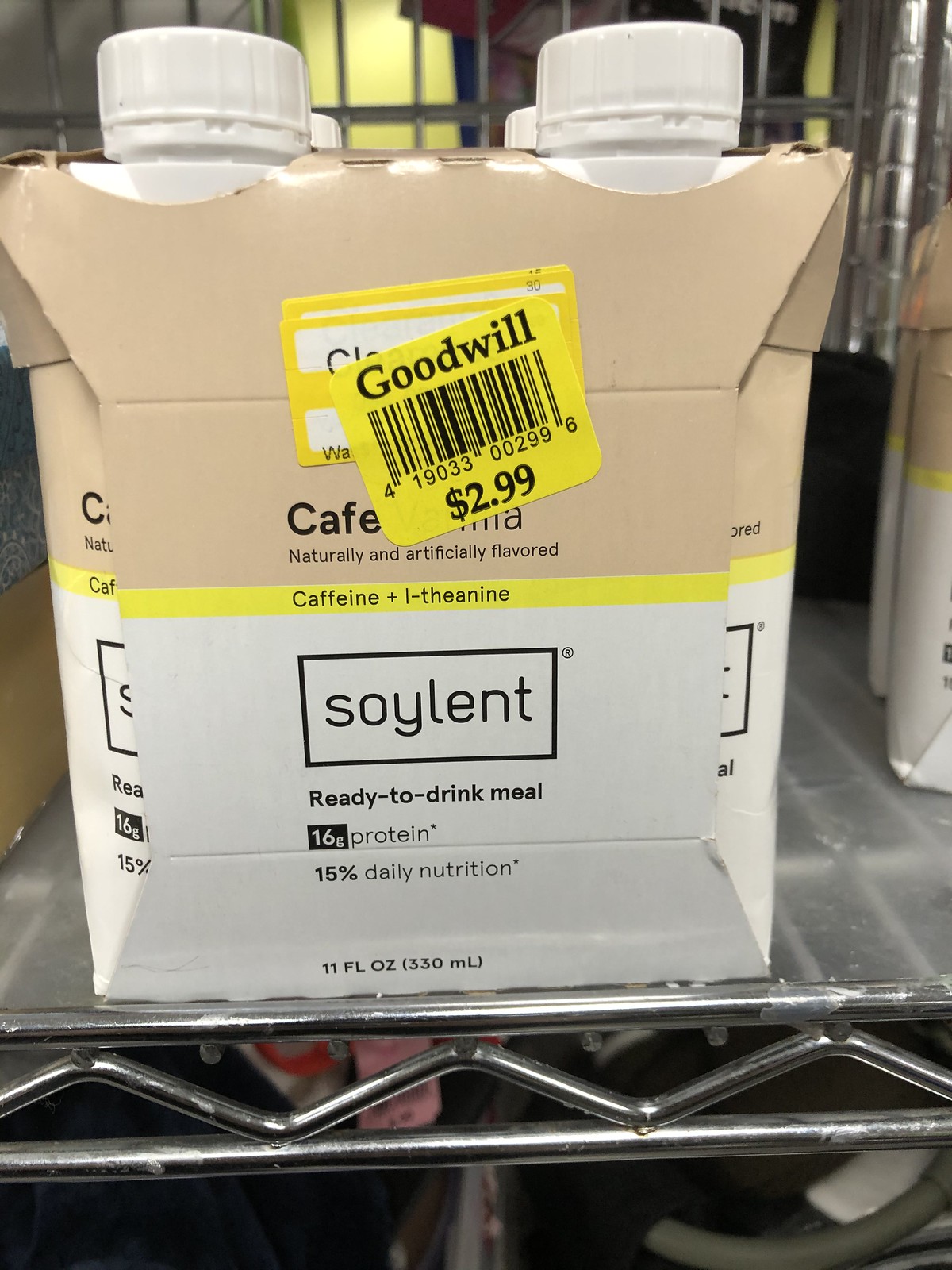In this image, we observe a product displayed on a chrome wire-type rack at a Goodwill store. The product is a four-pack of a nutritional drink, packaged in a carton that features a light brown color on the top half and white on the bottom half. The product's brand name, "Soyin," is prominently displayed on the carton. Additionally, a thin yellow line on the packaging highlights the presence of caffeine and theanine in the drink. Beneath the Soyin logo, the text reads "ready to drink meal," boasting 16 grams of protein and 15% of daily nutrition. A yellow Goodwill price tag is affixed to the carton, indicating the selling price of $2.99.